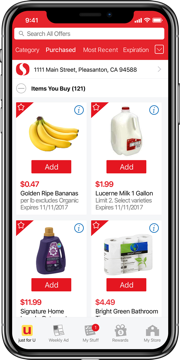This image features an AI-generated depiction of a shopping app on a cell phone. The cell phone appears to be a silver device, displayed in portrait orientation. The screen is framed with a red border at the top and a white background beneath it. The top red section is rectangular and houses vital information including the time, displayed as "9:41" in white, alongside icons indicating full network connectivity, Wi-Fi strength, and battery life, all also in white.

Beneath this red bar is a prominent search bar. It's white with a gray magnifying glass icon and the text "Search All Offers" in gray font. There are several selectable options below this search bar in gray text: Category, Purchased, Most Recent, and Expiration, accompanied by a drop-down arrow. The "Purchased" option is highlighted in white, indicating it is currently selected.

Underneath these options, there's a circular logo featuring a wavy white center with a red exterior. Next to this logo, the text reads "111 Main Street, Pleasanton, California" followed by the heading "Items You Buy," which has a minimized arrow indicator and the number "121" beside it, possibly indicating the number of items in a list.

Further down, the app lists some favorite items frequently purchased by the user, marked with stars in the upper left-hand corner of each item: Bananas, Milk, Laundry Detergent, and Paper Towels. These items are part of a banner displaying favorite selections, enhancing the user's shopping experience by allowing quick access to commonly bought items.